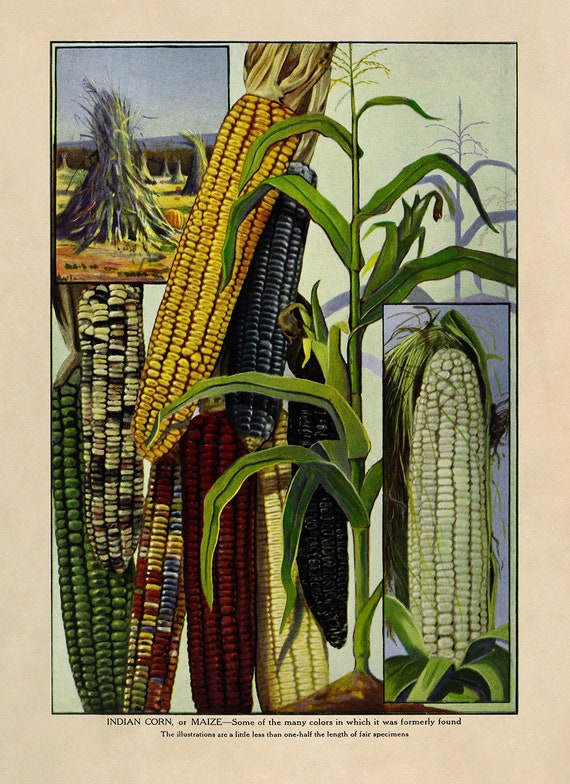The image is a detailed illustration showcasing various types of Indian corn or maize, each depicted in vibrant colors. The vertical rectangular picture features a tan border and contains a caption at the bottom that reads: "Indian corn or maize – some of the many colors in which it was formerly found. The illustrations are a little less than one-half the length of their specimens." The corn types are arranged in a visually appealing manner, with a dramatic yellow corn at the top, its husk pulled back. Beside it is a black variety of corn. Moving right, there is black corn transitioning into a lighter black, followed by solid red corn, mixed-color corn with yellow, blue, and red kernels, and green corn on the left. Additionally, there is a smaller, almost white corn. The image captures the diversity of the corn varieties, with each cob displaying distinctive hues such as pale yellow, solid yellow, black, red, and multicolored. In the background, various plant stems are visible, enhancing the natural and vivid portrayal of these historically significant corn types. The lighting is bright and natural, highlighting the intricate details of the illustrations.